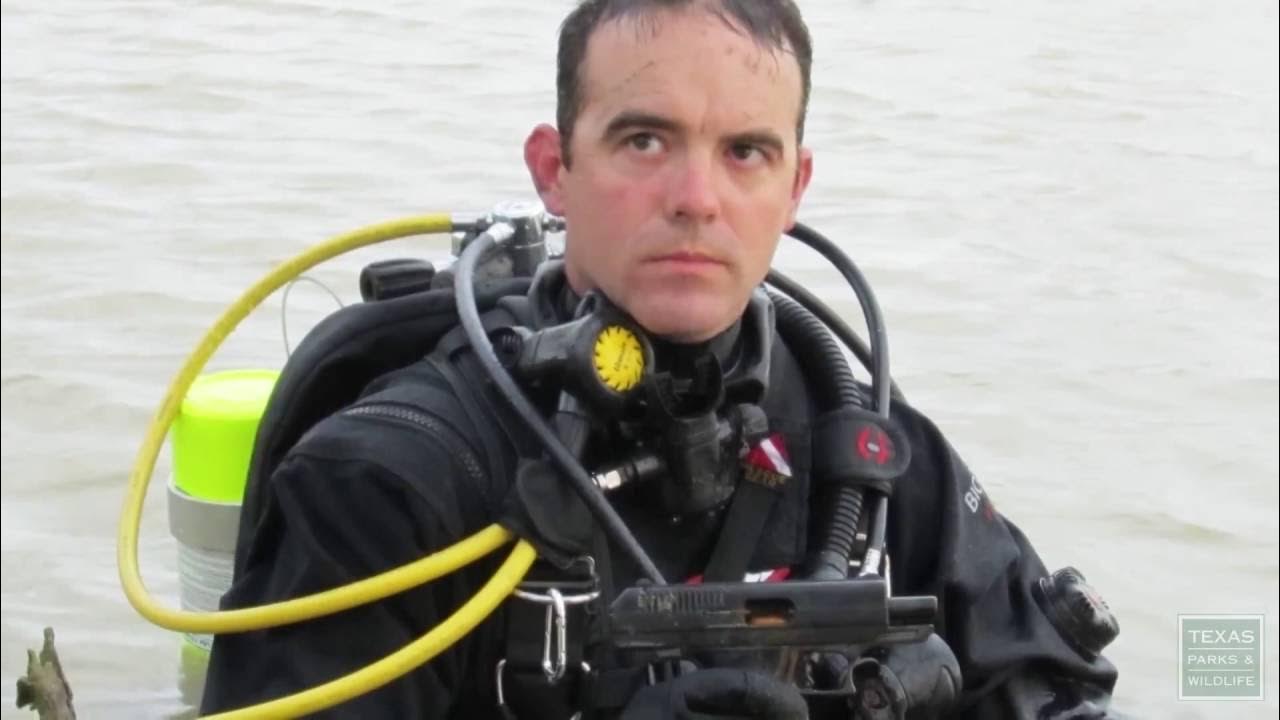This detailed photograph, potentially a screenshot from a video, showcases a diver at the center, half-submerged and emerging from a body of water that could be a river or lake. The diver, a man with a short, slightly disheveled haircut, is equipped with a black wetsuit and a yellow-and-clear air tank on his back. Numerous tubes, including bright yellow and black ones, extend from the tank to his gear. Notably, he is without a headgear, mask, and mouthpiece, which have been removed. In his hand, he holds a small, rusty handgun, nearly blending in with his dark wetsuit. The diver appears alert, looking up at someone, suggesting a sense of awareness to his surroundings. In the bottom right corner, the image features the text "Texas Parks and Wildlife" in white lettering on a gray box with a white outline.